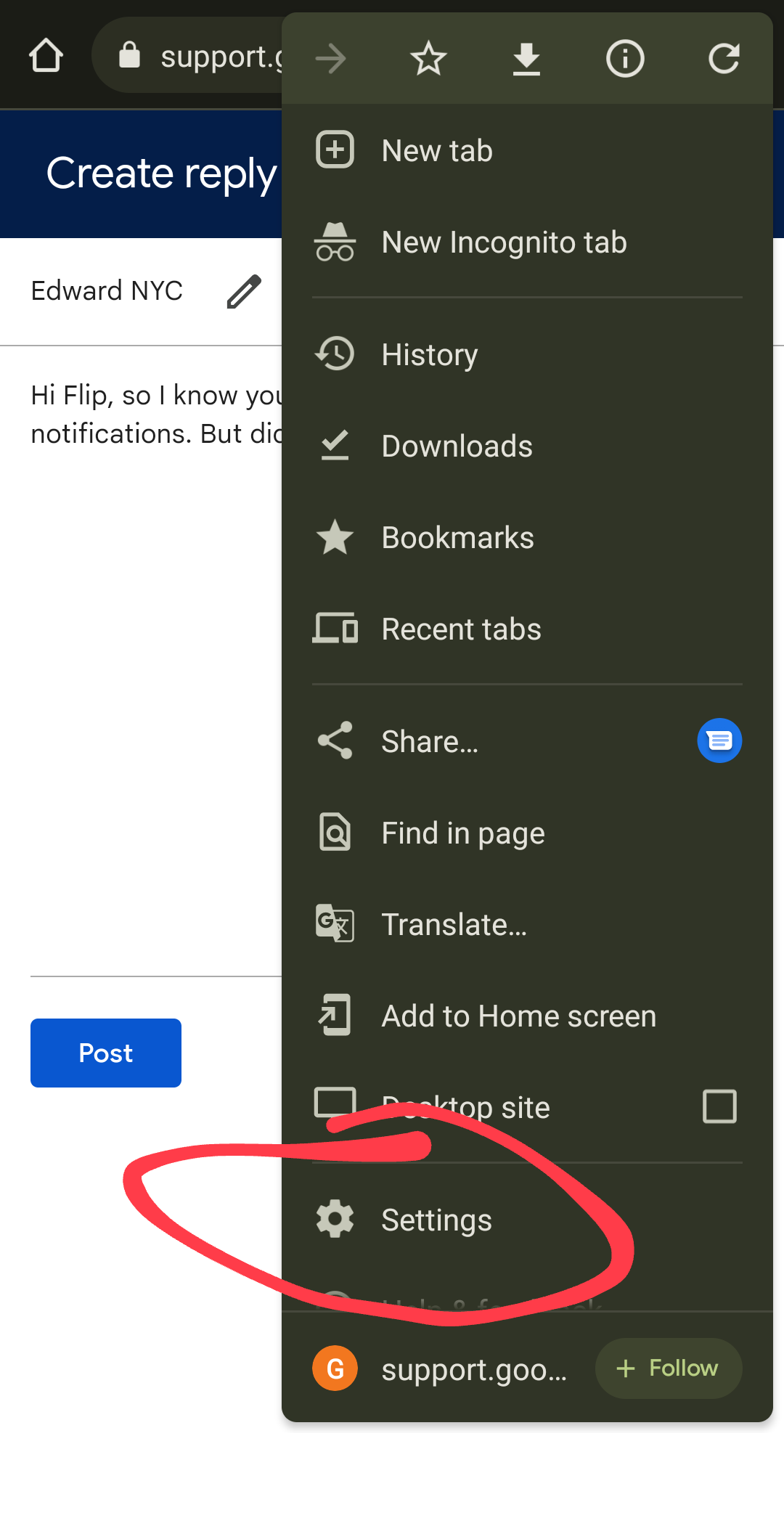The image depicts a smartphone screen showing a website with a detailed interface. On the right side of the screen, there is a prominent pull-out menu that appears brown or green in color. This menu contains numerous options, including "New Tab," "New Incognito Tab," "History," "Downloads," "Bookmarks," "Recent Tabs," "Share," "Find in Page," "Translate," "Add to Home Screen," and "Desktop Site." A "Settings" option, accompanied by a cog icon, is highlighted with a large red hand-drawn circle, suggesting it was marked for emphasis.

At the bottom of the menu, there's a notable red "G" icon representing Google, along with a message that reads "Support Google," and a small "Follow" button indicated by a plus sign. On the left side of the screen, there's a sizable blue "Post" button and a home icon. The phrase "Create reply Edward NYC" appears, though partially obscured by the pull-out menu, alongside a blocked-out message, indicating the presence of additional content underneath the tabs.